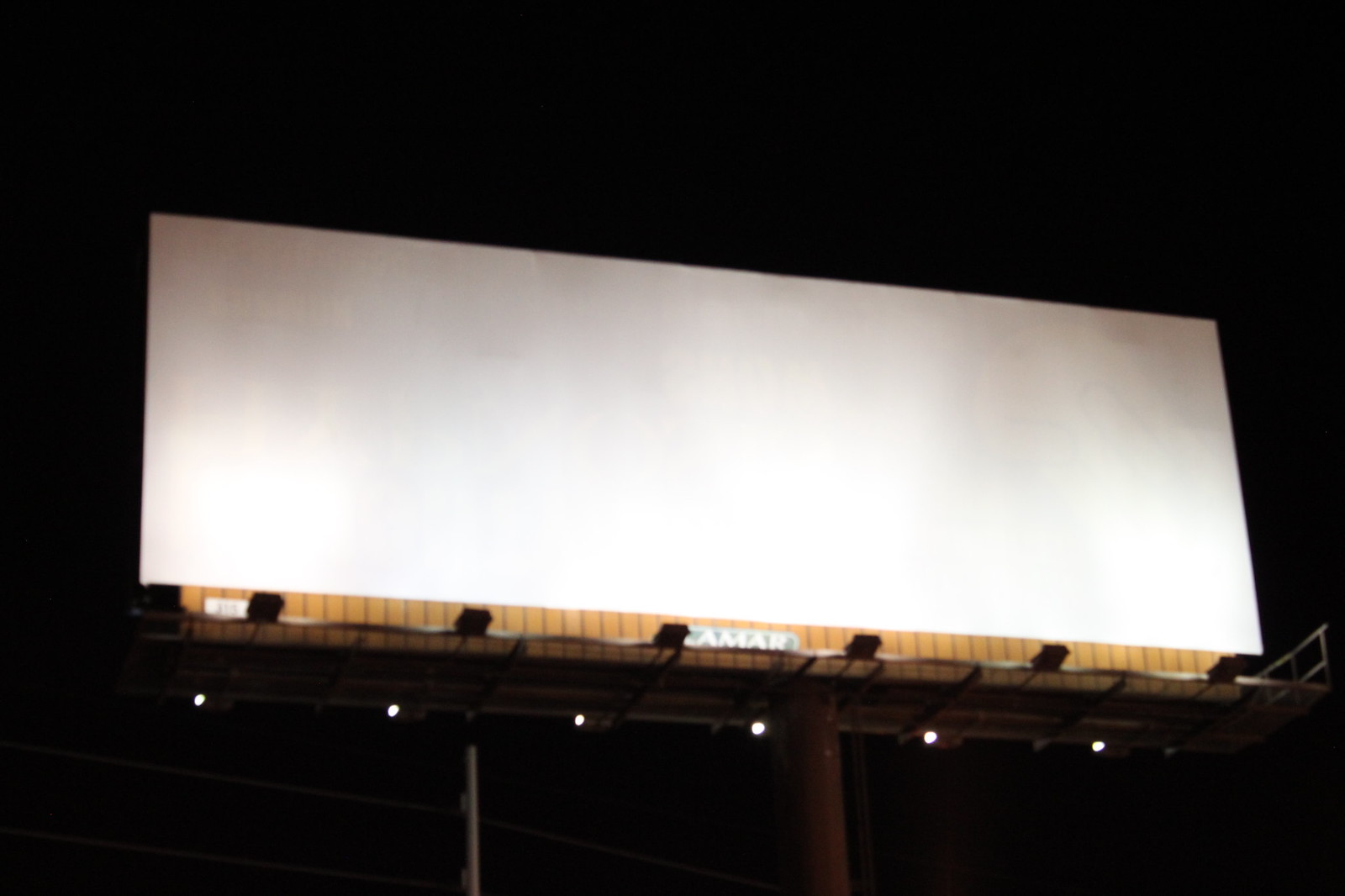The photograph captures a large, rectangular billboard set against a night sky, indicated by the black background. The billboard, suspended by two brownish, rust-colored poles, is completely blank and white with no advertisements on it. Shadows are prominently cast across its surface. The lower edge of the billboard features a brown or orange border, possibly as part of its structural support. Beneath this border, the label 'Lamar' is visibly displayed in green text with white writing. Illuminating the billboard are six lights positioned along the bottom, casting beams upwards. The black background hints at the photo being taken outdoors at night, enhancing the shadows and the overall contrast of the scene. Electrical lines are faintly visible under the left side of the billboard, further contributing to the intricate details of the nighttime setting.